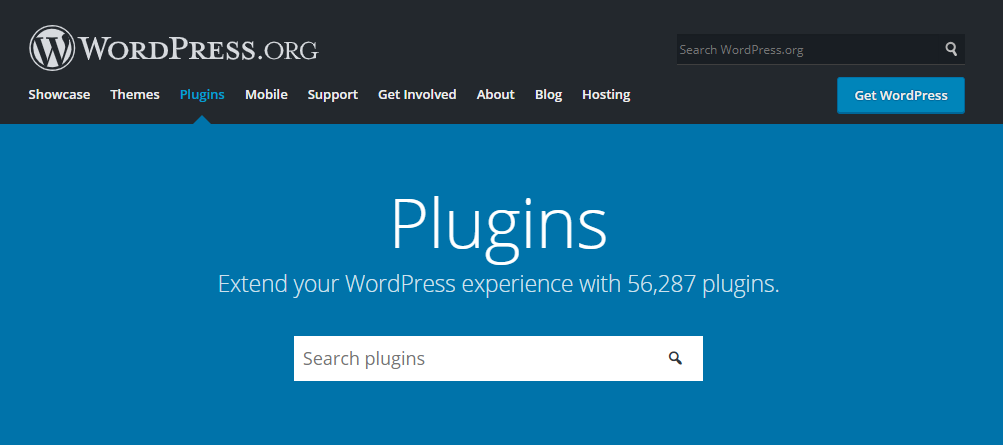The image depicts a section of the WordPress.org website. At the top-left corner, the WordPress.org logo is prominently displayed, consisting of the name "WordPress.org" in white text accompanied by a circular emblem featuring a black letter "W" on a white background. On the top-right corner, there is a search bar with the placeholder text "Search WordPress.org" and a white magnifying glass icon at its far right.

Below the header, there is a horizontal navigation menu with several categories listed from left to right: Showcase, Themes, Plugins (highlighted in blue to indicate it is currently selected), Mobile, Support, Get Involved, About, Blog, and Hosting. Towards the far right of the navigation menu, a blue rectangular button labeled "Get WordPress" is visible.

In the central part of the image, the word "Plugins" is prominently displayed, followed by a tagline that reads "Extend your WordPress experience with 56,287 plugins." Directly below this tagline is another search bar designed for users to search for specific plugins, featuring the placeholder text "Search plugins."